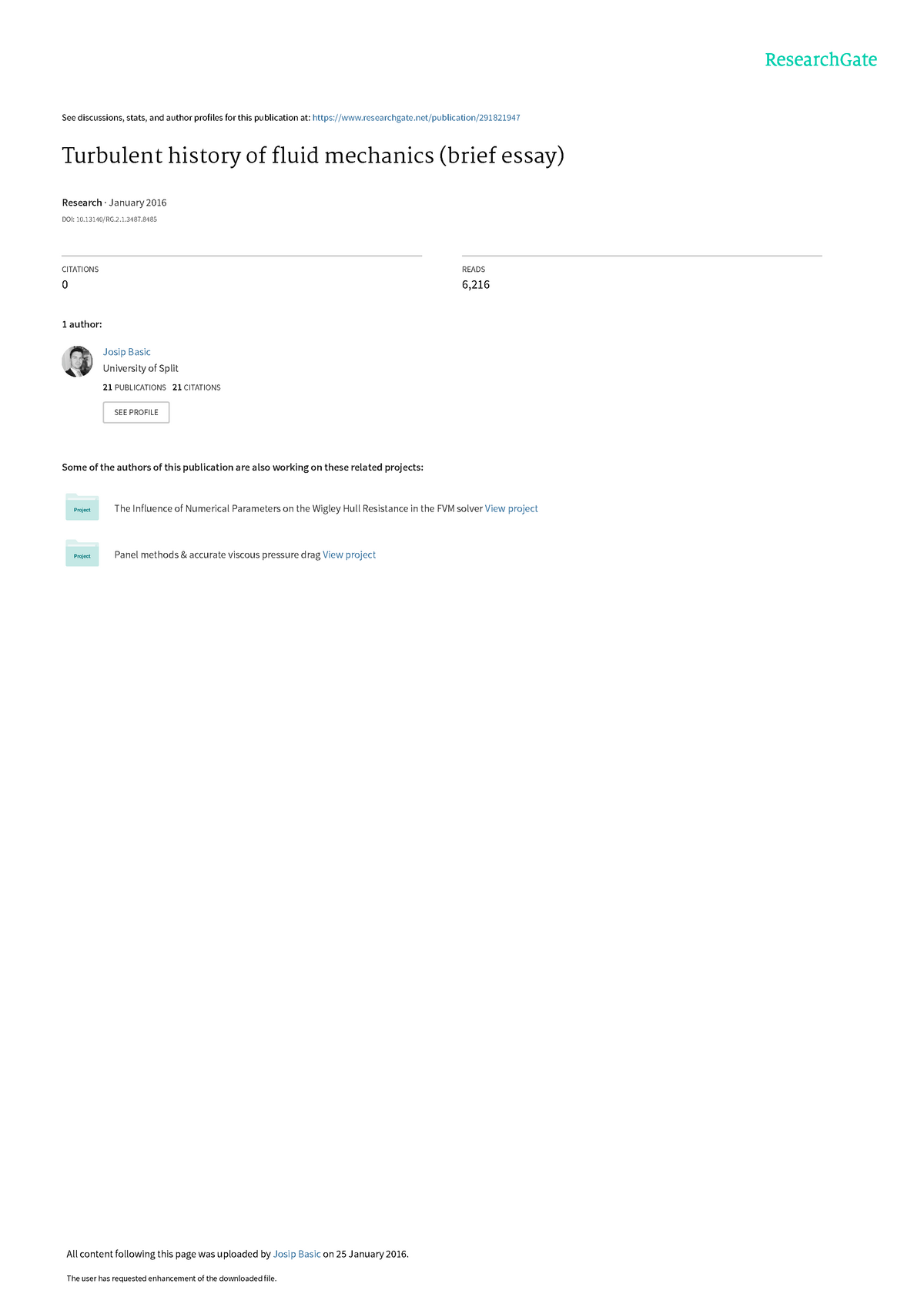An image capturing a section of a web page, likely from ResearchGate, featuring an article titled "Turbulent History of Fluid Mechanics (Brief Essay)." The interface is minimalist with a white background and most text rendered in tiny, nearly illegible fonts. In the top right corner, "ResearchGate" is prominently displayed in turquoise. Centered on the screen, the article title is the most readable element, accompanied by a small thumbnail image of a man, presumably the author, affiliated with a university—though the exact institution name is unclear. Additional text below the title features a January 2008 publication date and possibly includes the author's name and other metadata, but the text is too small to discern. Below this section, there are links to two more articles, similarly tiny and unreadable, with the bottom of the page displaying some copyright information, closing out the sparse layout.